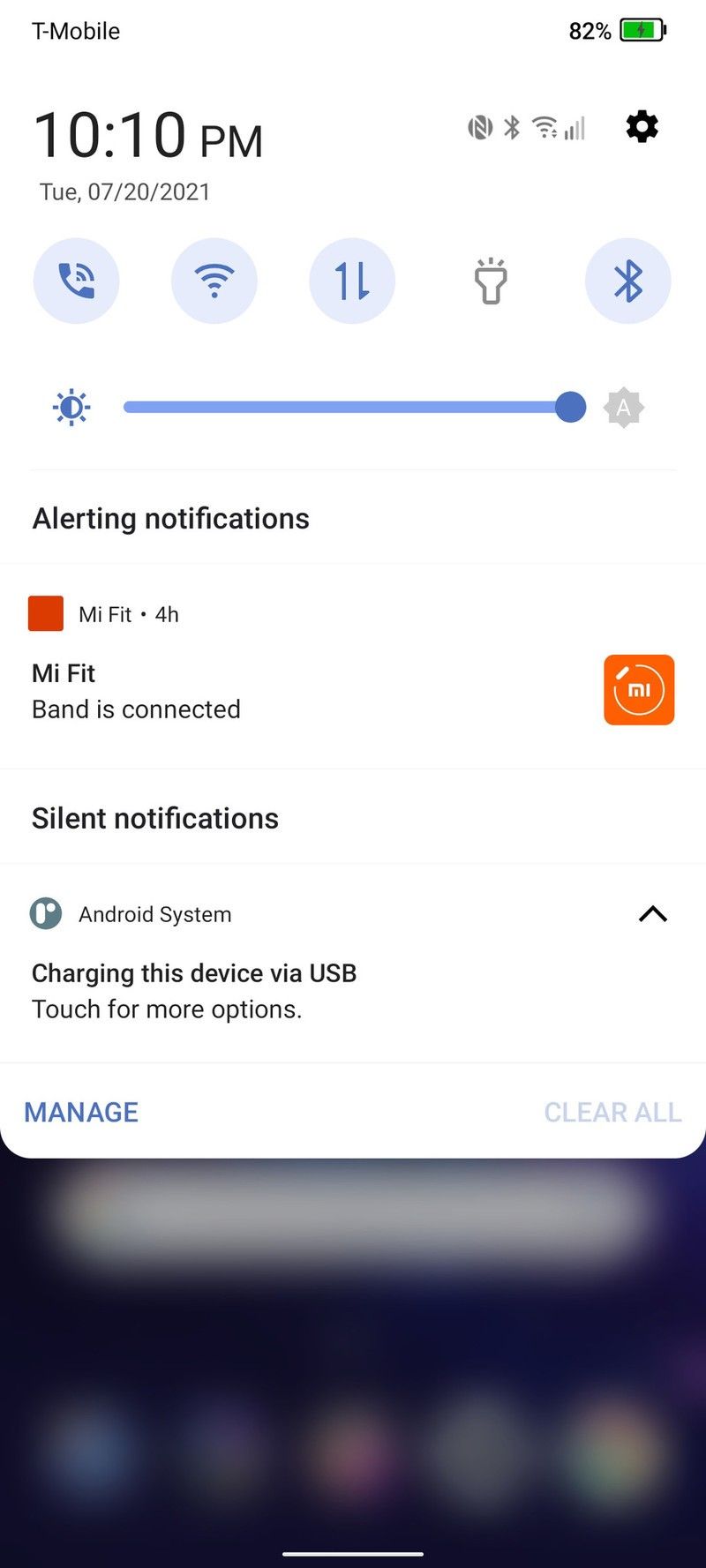In this detailed image, we see a screenshot of a cell phone display set against a pristine white background. At the top left corner, the screen indicates the network provider "T-Mobile" in bold black text. On the upper right side, a battery icon shows a charge level of 82%, and it's immediately flanked by icons signifying Wi-Fi connectivity and settings. The time is prominently displayed at "10:10 PM" just beneath the T-Mobile text. Further to the right, the date is presented as "Tuesday, 7-20-2021."

Just below these details, a blue circular icon is visible, indicating an active phone ringer, alongside icons for Wi-Fi and a flashlight function. Directly beneath these icons, there's a brightness control bar, positioned towards the extreme right to suggest maximum screen brightness.

Continuing downwards, a section titled "Alerting Notifications" appears in black text, followed by a notification from the "MyFit" app confirming that a band is successfully connected. Below this is another section labeled "Silent Notifications," where the "Android System" notification can be seen, providing information about the device being charged via USB with an option to touch for more details.

Finally, the lower portion of the screen transitions into a black rectangular area devoid of additional visual elements.